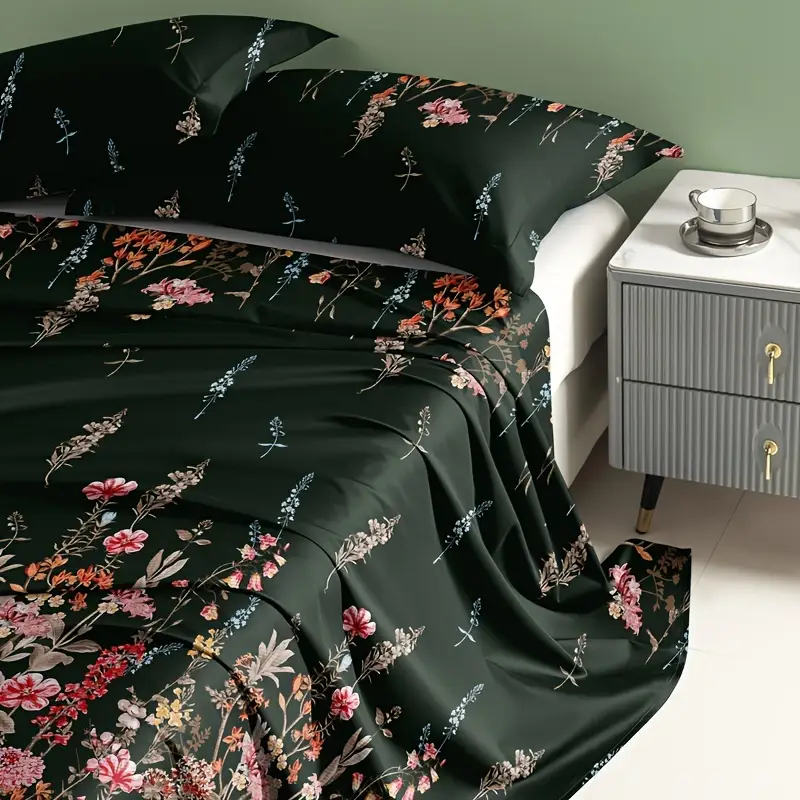The photograph captures a cozy corner of a bedroom featuring a stylish bed and an accompanying nightstand. The bed, dressed in a combination of intricate and plain designs, showcases a plain white sheet beneath a wrinkled black bedspread adorned with a beautiful floral pattern reminiscent of a delicate Japanese kimono. This elegant design is also mirrored on the matching pillowcases that cover the two pillows positioned at the head of the bed. The floral pattern features warm hues of red, pink, and orange flowers set against a dark green background, adding a touch of exotic charm to the room. The headboard is not visible; instead, the light sage green wall behind the bed softly complements the vibrant bedding.

Next to the bed stands a gray nightstand with two drawers distinguished by golden latches, adding a touch of sophistication. The top of the nightstand is white and serves as a resting place for a metallic, silver-colored teacup and saucer, exuding a sense of elegance and tranquility. The entire scene is grounded by a clean, white-tiled floor, contributing to the crisp, serene ambiance of the bedroom. Only the top right corner of the bed is visible in the image, suggesting a mid-sized and inviting sleeping space perfect for two.